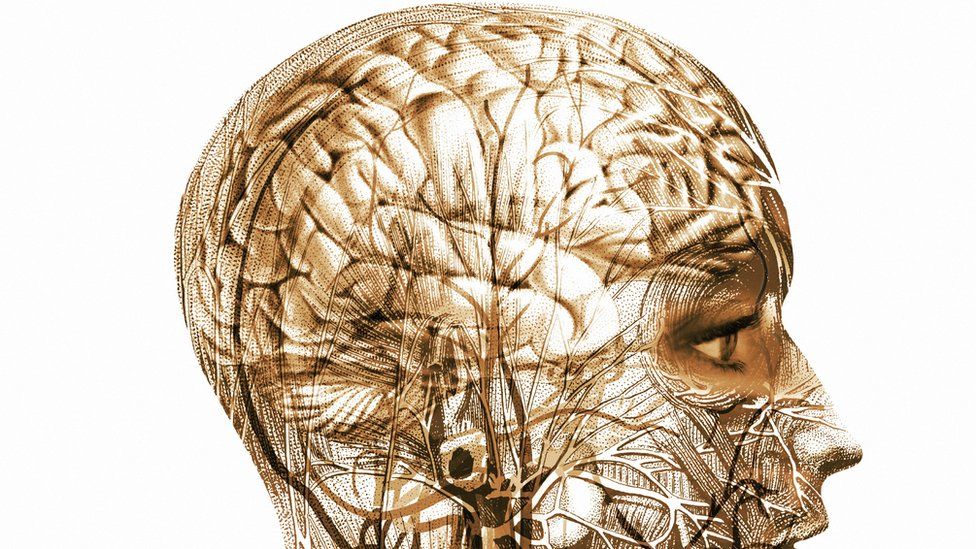This image is a digitally layered, sepia-toned illustration with a white background, depicting the intricate anatomy of a woman's head. The profile view reveals an extensive overlay of anatomical details including a highly detailed photorealistic eye with long eyelashes, and faintly visible nostril and top lip. The woman's head appears transparent, exposing various internal structures such as veins, muscles, and an unusually detailed brain with visible curves and folds. Dark shadows and varying shades of brown emphasize the different anatomical features, with veins and neural pathways intricately mapped out. The composition is further complicated by an overlay of fine, thin branches resembling a tree, adding to the overall complexity and depth of the image. While the detailed depiction of the brain, eye, and neural pathways stands out, the layering and transparency create a visually elaborate and somewhat confusing presentation.